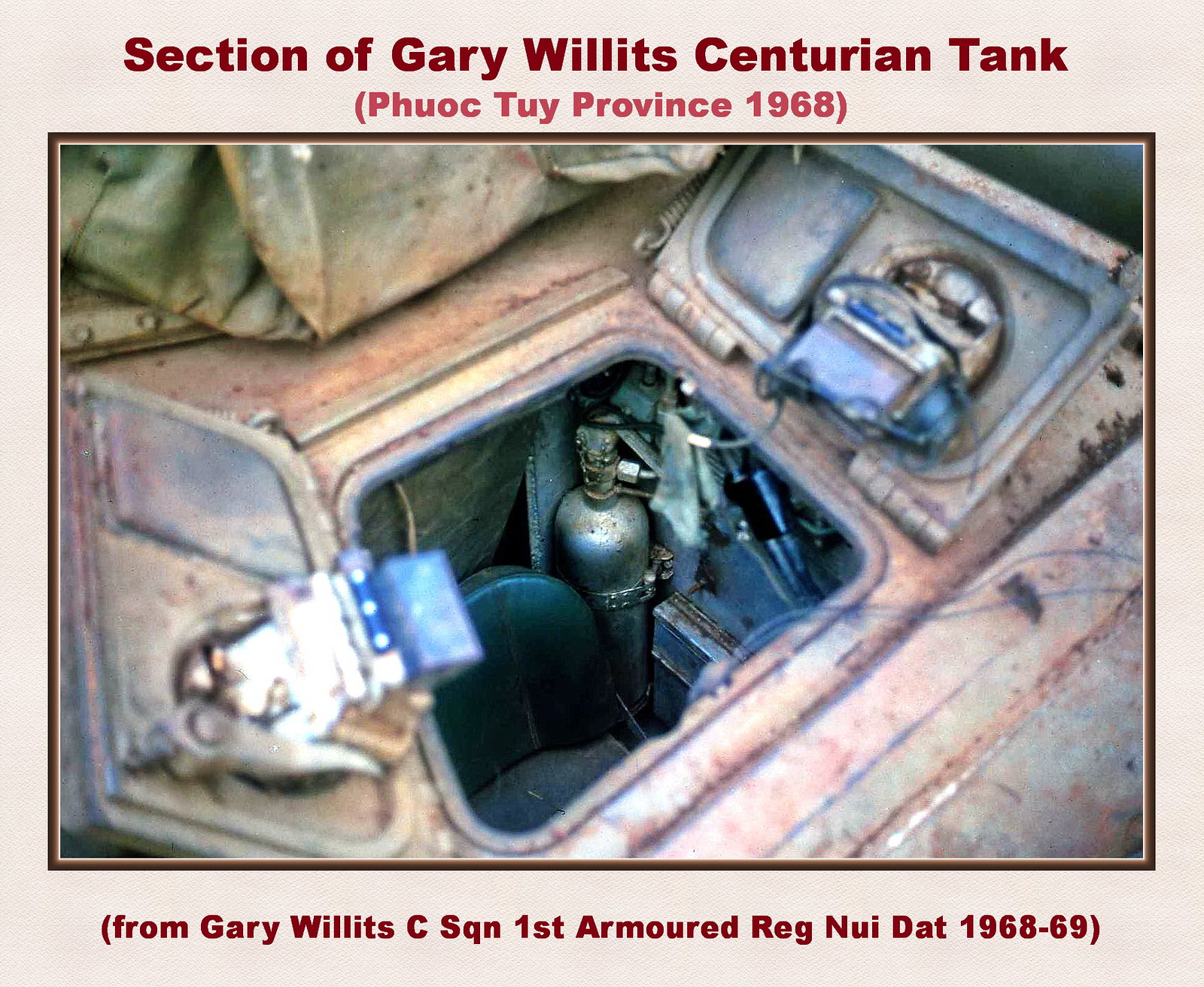This image, bordered by a combination of colored frames, features an intricate glimpse into the interior of a military vehicle from the Vietnam War. The outermost border is cream-colored, succeeded by a brown border enclosing the photograph. At the top, in dark red text, it reads "Section of Gary Willits' Centurion Tank." Just below it, in a lighter red, is indicated "(Phuoc Tuy Province, 1968)." At the bottom, in similar dark brownish-red text, it is noted "(From Gary Willits, C-Squadron, First Armored Regiment, Nui Dat, 1968-69)." The focal point of the image is the open hatch of the tank, revealing its interior. The hatch, with two doors open on either side, exhibits a light brown hue. Inside, a small black seat is visible, alongside what seems to be an oxygen tank secured by metal latches. Additional elements such as a metal canister and a green tarp are also discernible within the cockpit area. The exterior and visible components of the tank display varying shades of light brown and pink, contrasting with the utilitarian, metallic interior.